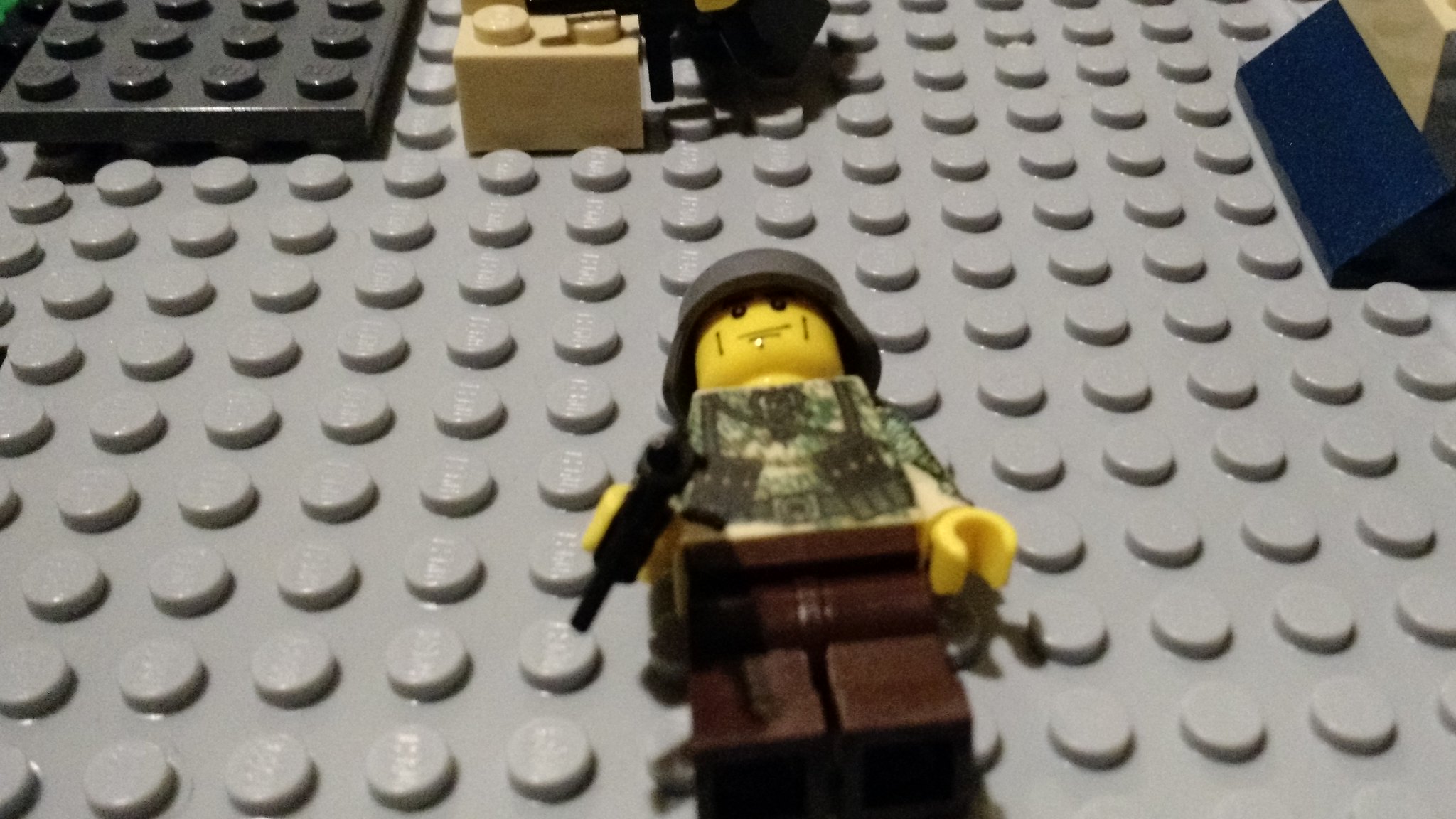The image depicts a slightly blurry and poorly lit scene featuring a Lego military figure laying on its back on a large, flat, gray Lego board with the typical raised convex points. The figure, resembling a soldier, has a yellow face and hands, a dark gray helmet, a camouflage-printed torso with what appears to be detailed military gear, and brown legs. The soldier, seemingly holding a black gun in its right hand, also has what looks like a cigarette in its mouth. This figure is positioned at the center of the photo with its feet towards the camera. Scattered around the gray Lego base are other pieces, including a flat horizontal black piece and a light off-white piece. In the distant background, another Lego character can be seen, contributing to what looks like a battlefield-themed Lego setup.